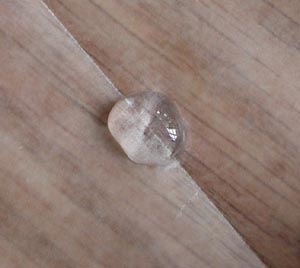The image features a light beige backdrop with a surface resembling wood, marked by fine vertical gray or brown lines and mottled brown patches. A noticeable diagonal crease runs across the image from the left-hand corner to the right-hand corner. Resting at the center of this crease is a clear, transparent water droplet or fluid oval, which appears lumpy and liquidy. The droplet's clarity reveals no inherent color, creating an impression of a transparent stone or valuable gem. The textured, wood-like surface beneath enhances the visual contrast with the droplet's glossy, smooth texture.